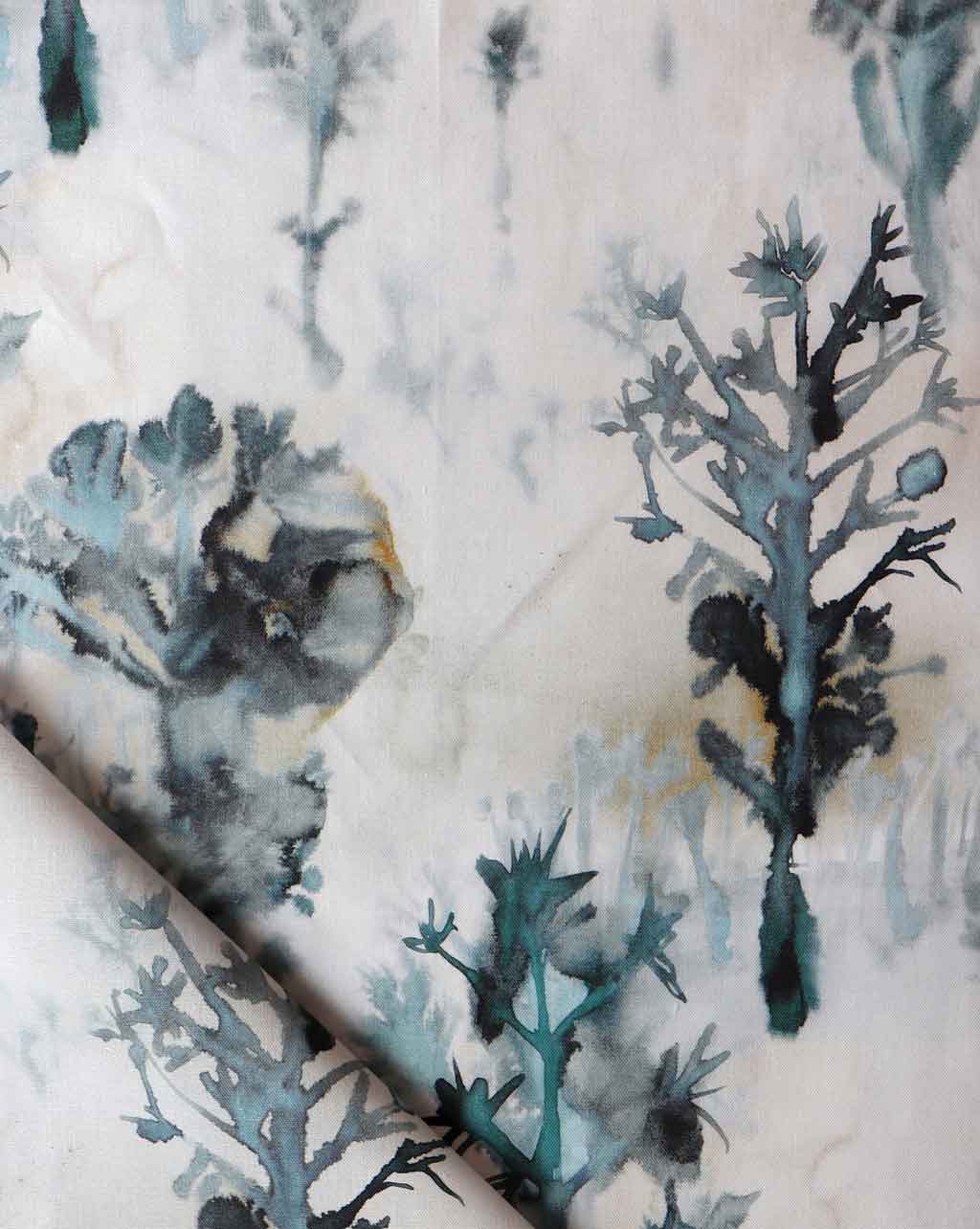The image features an abstract painting set against a predominantly gray background with subtle infusions of blue and green. The textured backdrop evokes the look of watercolor, with colors seamlessly fading into one another. Dominating the foreground are tree-like structures, reminiscent of Joshua trees or cactuses, painted in shades of midnight green, turquoise blue, and dark blue-black. These forms stretch across the left, right, and bottom of the composition, with some branches appearing faint and blurred, giving the impression of depth and distance. Interspersed among these primary elements are patches of brown and orange, possibly resembling stains or highlights, further enhancing the rustic feel. The bottom part of the painting has a noticeable crease that runs from the left edge towards the middle, adding an element of texture and imperfection to the artwork.